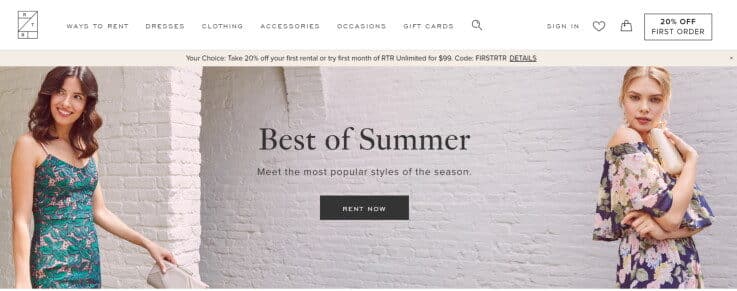This screenshot captures the homepage of a fashion rental website. In the upper left-hand corner against a white background, there is a rectangular logo featuring a diagonal line running from the bottom left to the top right, intersected by horizontal lines at the top and bottom, and some embedded letters.

The top menu bar, set against a gray background, spans the width of the page and includes the options: 'Ways to Rent,' 'Dresses,' 'Clothing,' 'Accessories,' 'Occasions,' and 'Gift Cards.' A gray magnifying glass icon for the search function is to the right of these options. Additionally, there are three icons to the right: a 'Sign-In' button, a purse outline, and a gray-outlined rectangle highlighting a '20% off first order' promotion.

Directly below the menu bar is a horizontal promotional banner. The top edge of this banner features a beige strip with black text. The banner is divided into three sections. On the left, there is an image of a woman with long dark hair wearing a spaghetti strap dress with a green and beige print, posing against a white painted brick wall. The center of the banner features the text "Best of Summer" in black, with a black rectangular button below that says "Rent Now." On the right side, another woman with blonde hair pulled up is depicted. She is wearing an off-the-shoulder dress adorned with green, beige, and pink floral patterns.